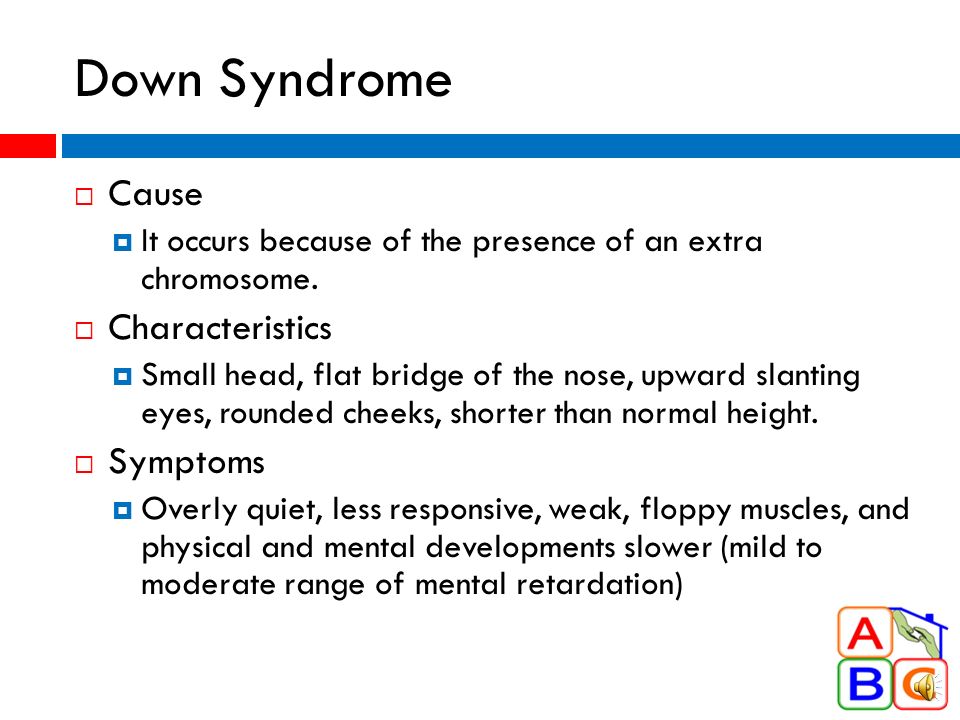The web page about Down syndrome features a stark white background with black text, ensuring clarity and readability. At the top left corner, prominently displayed in large letters, is the title "Down Syndrome." Directly beneath the title is a horizontal bar, characterized by a small red segment on the left and a dominant blue portion extending across the rest of the bar.

Below this visual banner, the section titled "Cause" appears, indicated by a small red square to its left. Adjacent to a small blue square, the detailed cause is explained: "Down syndrome occurs because of the presence of an extra chromosome."

The next section, "Characteristics," is also marked with a red square, and the subsequent detailed list, indicated by a blue square, includes: small head, flat bridge of the nose, upward slanting eyes, rounded cheeks, and shorter than normal height.

Following this, the section "Symptoms" is introduced with another red square, with the descriptive list marked by a blue square. The symptoms include: overly quiet demeanor, less responsiveness, weak and floppy muscles, slower physical and mental development, and a range of mild to moderate cognitive impairment.

At the bottom right of the web page, the website’s logo is displayed. This logo consists of three blocks: the top left block contains the letter "A," the bottom left block contains the letter "B," and the bottom right block contains the letter "C." There is also a nearly complete block in the top right corner, resembling the corner of a house's roof.

This structured, color-coded layout ensures that information about Down syndrome is both comprehensive and easily navigable.